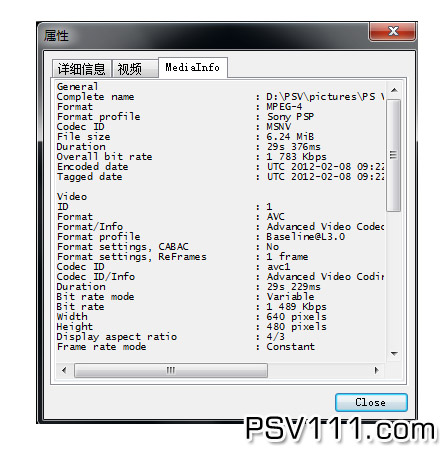This image is a screenshot of a Windows application window displaying media information. The window has a typical Windows interface with a red X button at the upper right corner to close it. In the upper left corner, prominently displayed, are two characters in either Japanese or Chinese script. Beneath these characters are three tabs; the first two are labeled with Japanese or Chinese characters, while the third tab, selected and visible, is labeled "Media Info."

The Media Info tab displays an array of detailed information about a media file. On the left column, categories listed include General, Complete Name, Format, Format Profile, Codec ID, File Size, Duration, Overall Bit Rate, Encoded Date, Tag Date, Video ID, Format, Format Info, Format Profile, Format Settings (CABAC and Re-Frames), Codec ID, Duration, Bit Rate Mode, Bit Rate, Width, Height, Display Aspect Ratio, and Frame Rate Mode. The right column contains corresponding data for each category, with examples like MPEG-4, Sony PSP, and specific video dimensions (640 pixels by 480 pixels), durations, and bit rates.

At the bottom of the window, there's a slider bar indicating more information can be viewed by sliding left or right. Additionally, there's a "Close" button in the bottom right corner for exiting the window, and overlaid text at the bottom right reading "psv111.com." The whole interface is encapsulated within a black border, emphasizing its isolation from the surrounding desktop.